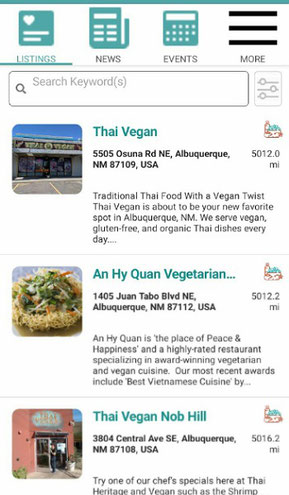This image depicts a slightly outdated screenshot from a phone, evident from the retro icons, the search bar, and the filter buttons that appear somewhat inconsistently placed and quickly designed. The screen displays a list of Southeast Asian vegetarian and vegan restaurants located in Albuquerque, New Mexico, USA. The restaurants listed include "Thai Vegan", "Anhee Kwan Vegetarian" (potentially also a Thai restaurant, although the pronunciation might be unclear), and "Thai Vegan Nob Hill". Accompanying each restaurant listing on the left-hand side are images: two showcasing the exteriors of the buildings and one featuring some food. The search results indicate that these restaurants are within a 5,000-mile range, possibly hinting that the search filters could be set to a broader scope potentially encompassing Thailand itself.